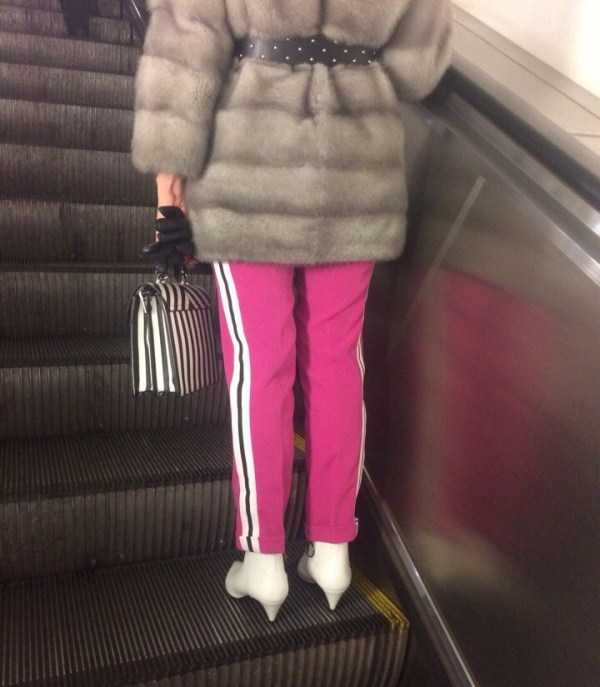The image captures a woman ascending an escalator, with the photo focused mid-back and extending downward, occupying the middle third of the frame. She's adorned in a dark gray, faux fur winter coat that extends below her hips, cinched at the waist with a black and white polka-dotted belt. Her left hand grasps a black and white striped handbag, along with a pair of black leather gloves. She wears pink sweatpants featuring outer side stripes in black and white, paired with white high-heeled boots adorned with gold buckles at the ankles. The escalator itself is typical in color, featuring silver interior walls, black stairs, and yellow edge markings on the steps.